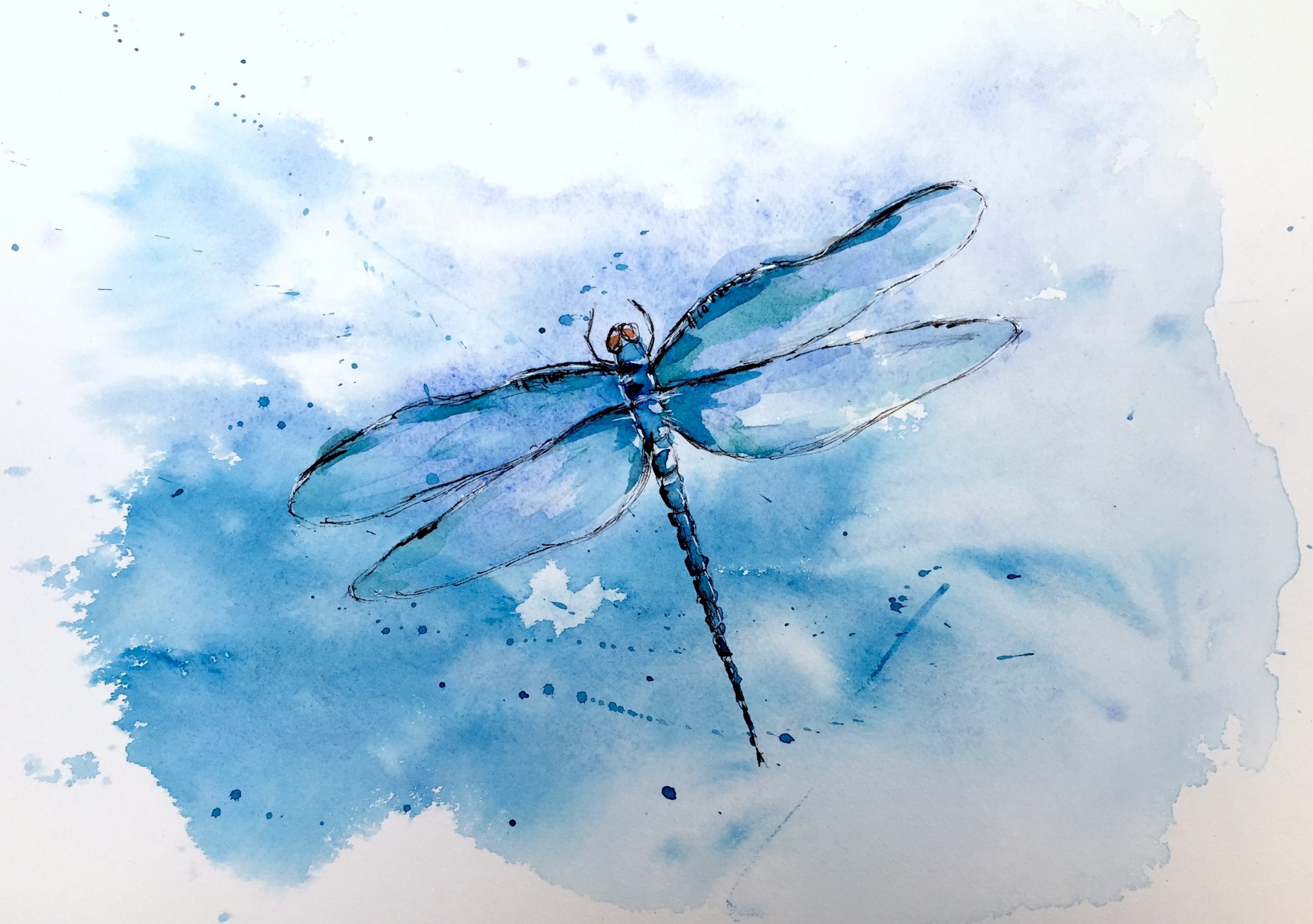This captivating watercolor painting features a blue dragonfly prominently displayed in the center, depicted from a top-down view with intricate details. The dragonfly, decorated in varying shades of blue, has segmented features including its body, head, back, and tail. Its four wings, delicately spread out to the sides, are highlighted with hints of light blue and purple and subtly outlined in black. The eyes of the dragonfly are depicted in a yellowish-orange hue. The painting's background is composed of an array of blue splotches, from dark to light, creating a striking contrast. The overall composition is enhanced by scattered droplets of darker blue paint, adding texture and depth to the scene. The dragonfly is slightly angled, pointing toward the 11 o'clock position, set against a mostly white and light blue background. This artistic piece is a simplified yet elegant representation of a dragonfly, showcasing the beauty of the watercolor medium.